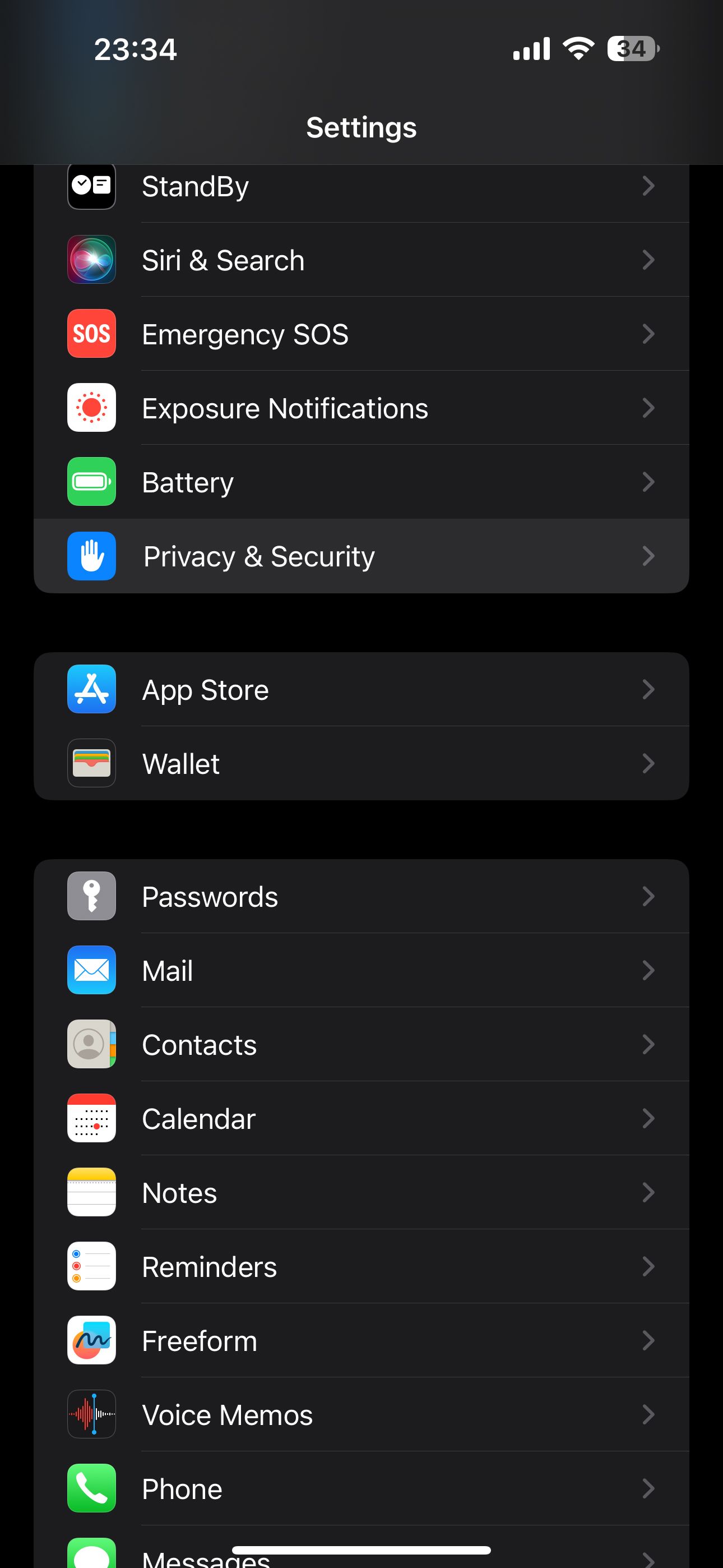The image displays the settings menu of an iPhone in dark mode, where the entire background is black. At the top of the screen, the time is indicated as 23:34, a Wi-Fi signal is shown to be connected, the battery icon reads 34%, and four bars signal cellular reception. 

The list of settings appears in white text, separated by thin white lines and accompanied by corresponding icons. The visible settings options include: 

- **Standby**
- **Siri & Search**
- **Emergency SOS**
- **Exposure Notifications**
- **Battery**
- **Privacy & Security**
- **App Store**
- **Wallet**
- **Passwords**
- **Mail**
- **Contacts**
- **Calendar**
- **Notes**
- **Reminders**
- **Freeform**
- **Voice Memos**
- **Phone**
- **Messages**

Each setting section is delineated with gray arrows indicating subsections. This detailed interface accurately represents the default layout seen when accessing the settings menu on an iPhone.